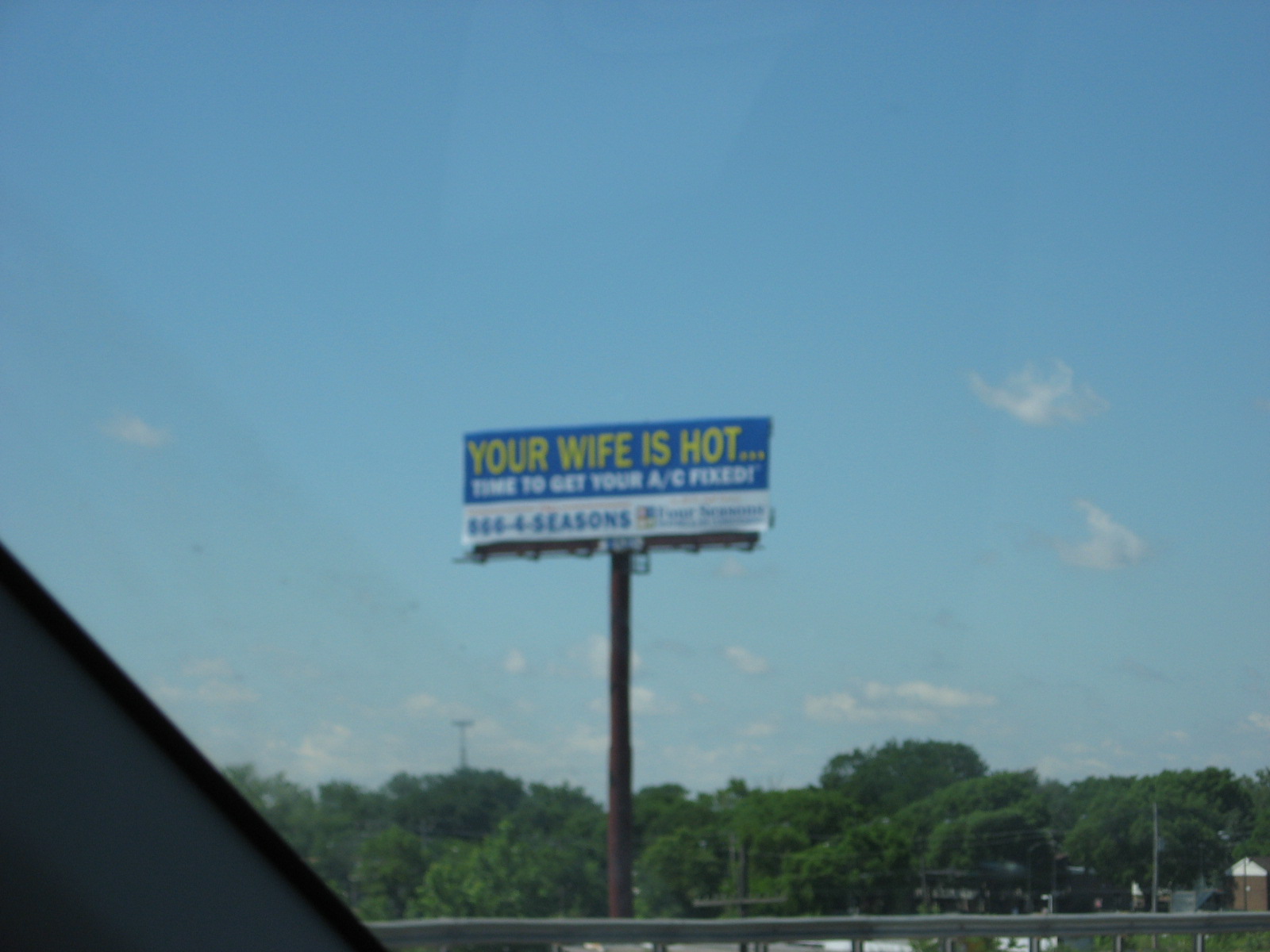A photograph captured from inside a car focuses on a large, rectangular billboard prominently displayed in the center. The billboard's upper section features a cheeky advertisement with bold, yellow text against a blue background stating, "Your wife is hot." Below this, white text reads, albeit blurry, "Time to get your AC fixed," creating a clever play on words to promote air conditioning services. The lower part of the billboard has a white background with a phone number and the words "Four Seasons," although some details here are also blurred. The billboard is mounted on a tall metal pole, positioned centrally in the image. The sky above is a clear blue with a few scattered white clouds, providing a cheerful backdrop. At the bottom of the image, a row of trees stretches horizontally, adding a natural element to the scene. The left edge of the photo includes a black triangular shape, likely part of the car's interior, such as the dashboard, entering the frame.